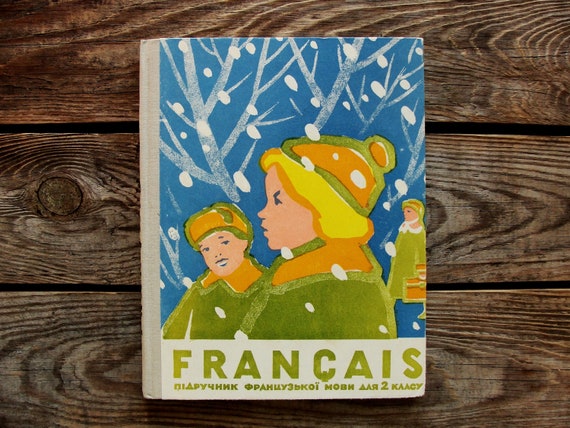This image features a highly stylized, colorful book cover laid on a dark brown wooden surface with slats. The cover illustration depicts three figures – a woman and a man in the foreground, and another woman in the background. All are wearing coats in various shades of green, paired with green and orange hats, amidst a backdrop of a blue sky with white tree branches and snow falling. The painting appears thickly textured, enhancing the visual appeal. At the bottom of the cover, the word "Francais" is printed in green, followed by what seems to be Russian text. The overall design suggests a fusion of languages and a wintery, conversational scene.